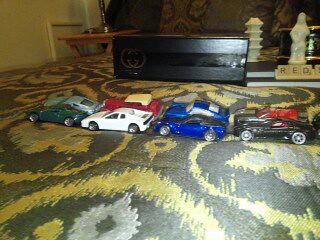The image depicts a detailed and colorful arrangement of eight miniature model cars on a gray and yellow rug with circular patterns. The cars are neatly lined up in a four by two formation, showcasing a variety of colors: directly facing front is a green car alongside a gray car. Behind them, a white car, resembling a miniature Corvette, is placed next to a red car. Further back, there are two blue cars, one with black windows and the other with gray, situated next to another black car. The setup is complemented by various objects in the background, including statues, Scrabble tiles spelling out the word "RED," and a black box that could be a VCR or radio transmitter. The scene appears to be inside a home, possibly with yellow lighting, representing a personal car collection displayed meticulously for the photograph.